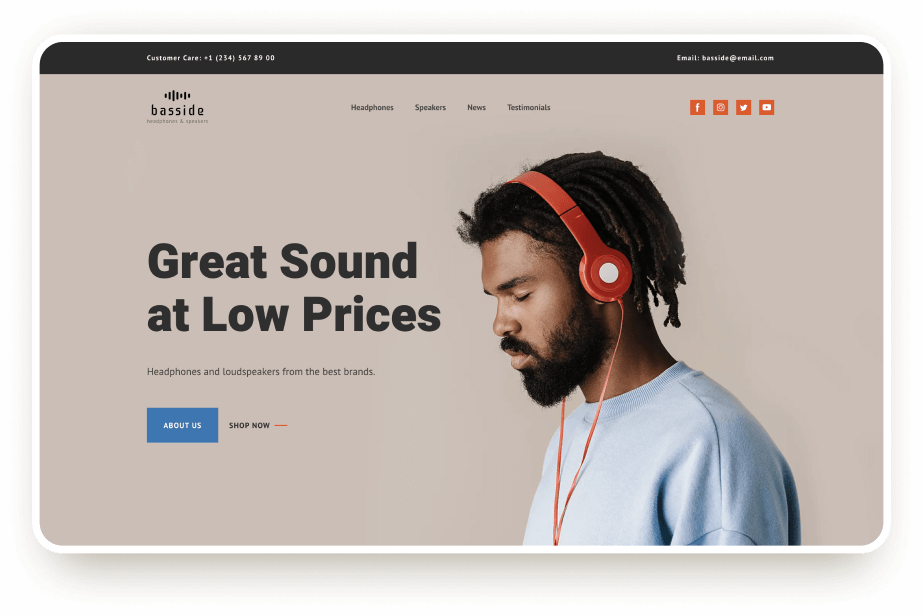The image depicts a webpage with a predominantly black background. 

At the top of the page is a header. In the top right corner, there is white text displaying an email address: "email@bathsite.com". On the top left, it says: "Customer Care: +1234 0000". Just below this, still on the left side, is a logo reading "Bathsite Headphones and Speakers," written in black on a light brown background.

Centered at the top of the page, there are navigation headers: "Headphones," "Speakers," "News," and "Testimonials," each in black text.

In the top right corner, there are four social media icons (Facebook, Instagram, Twitter, and YouTube) drawn in white on orange backgrounds.

In the center-left of the page, there is a prominent black text that reads: "Great Sound at Low Prices. Headphones and Loudspeakers from the Best Brand." Below this text, there is a blue button labeled "About Us," and to the right of the button is black text that says "Shop Now."

On the right side of the page, there is a picture of a person. This individual has black dreadlocks and is wearing a hooded blue jacket, with headphones on their head. The headphones are white and wired, with a red cable. The person's eyes are closed, and they are facing left.